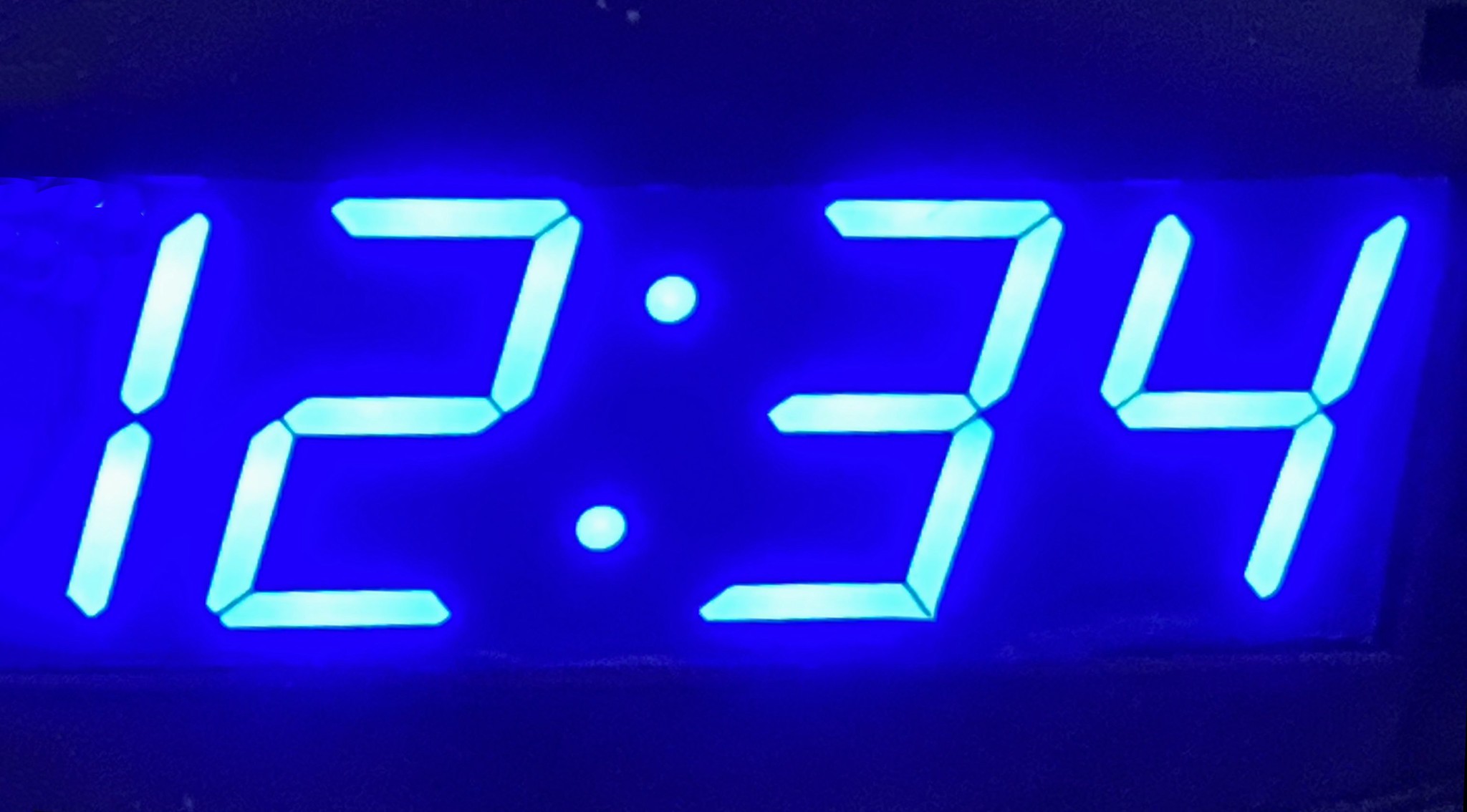This highly detailed close-up photograph captures a digital clock displaying the time "12:34." The image quality is commendable, though the intense neon lighting introduces a slight blur around the digits. These numbers glow in a radiant, neon blue hue, contrasting sharply with the darker blue background that remains vividly illuminated. The light from the clock seems to emanate and orbit around the numbers, adding a mesmerizing glow. Even the black space surrounding the clock appears tinged with blue due to the powerful brightness of the digits. The overall effect is a captivating blend of vivid neon and deep shadows.